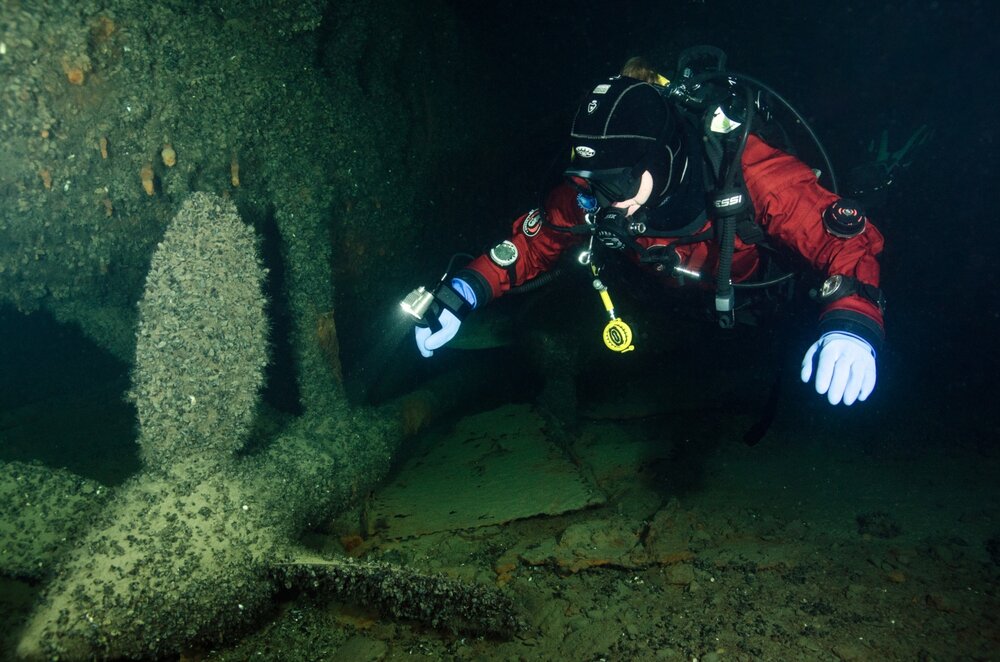This professional underwater photograph captures a deep-sea scuba diver, identifiable by a red wetsuit, white gloves, and a black helmet with attached black glasses, exploring what seems to be a shipwreck. Various yellow and green accessories are attached to the diver’s gear, which includes a flashlight affixed to their wrist. The diver stands on the seafloor, bathed in greens and yellows from the light and underwater vegetation. They are closely examining a large, algae-covered, metallic structure resembling a corroded ship propeller. This propeller, sitting amidst debris on the ocean floor, appears worn and ancient, signifying the prolonged underwater presence. The water is relatively clear, allowing for a detailed view of both the diver and the encrusted marine artifact, suggesting an environment rich in underwater life and history.